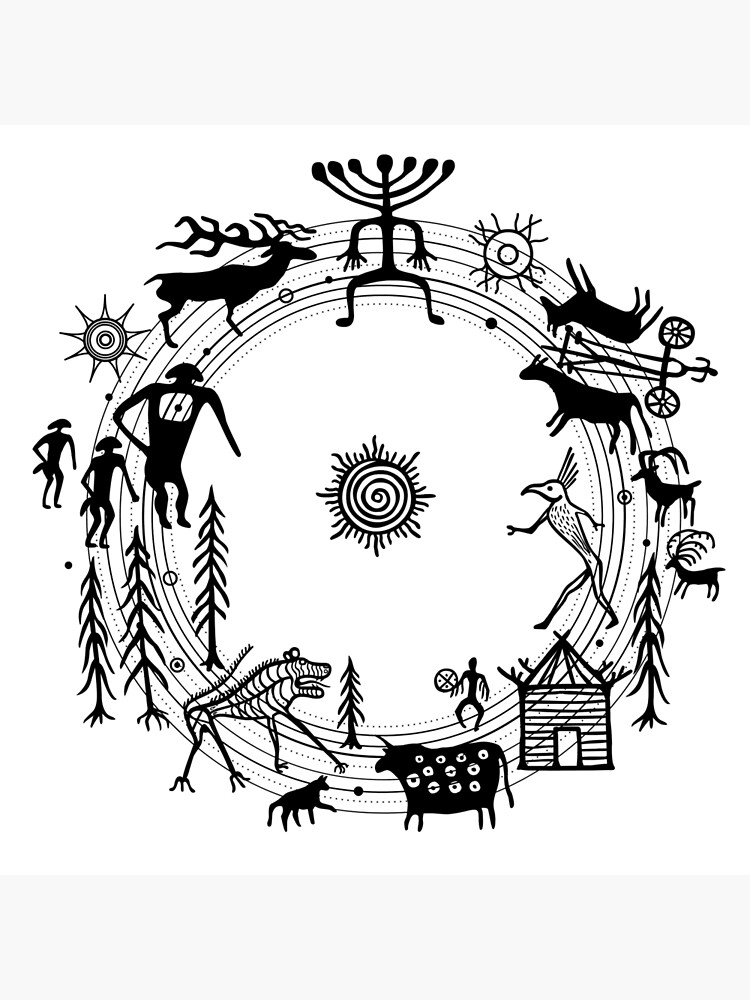The image features a detailed black and white ring-shaped design on a white background, evocative of primitive rock paintings. Central to the composition is a swirling sun surrounded by both solid and dotted circular lines. Within this intricate layout are various symbolic illustrations, including animals such as a reindeer, elk, bison, wolves, and a cow. Human-like figures appear amidst these, resembling tribal or caveman representations. Also included are tall, skinny trees and a small shed-like structure. Prominently at the top center, there is a unique figure that combines a human body with a candelabrum-like head branching out into multiple smaller heads. The design is rich with diverse symbols, giving it a primitive, almost mythological universe aesthetic.